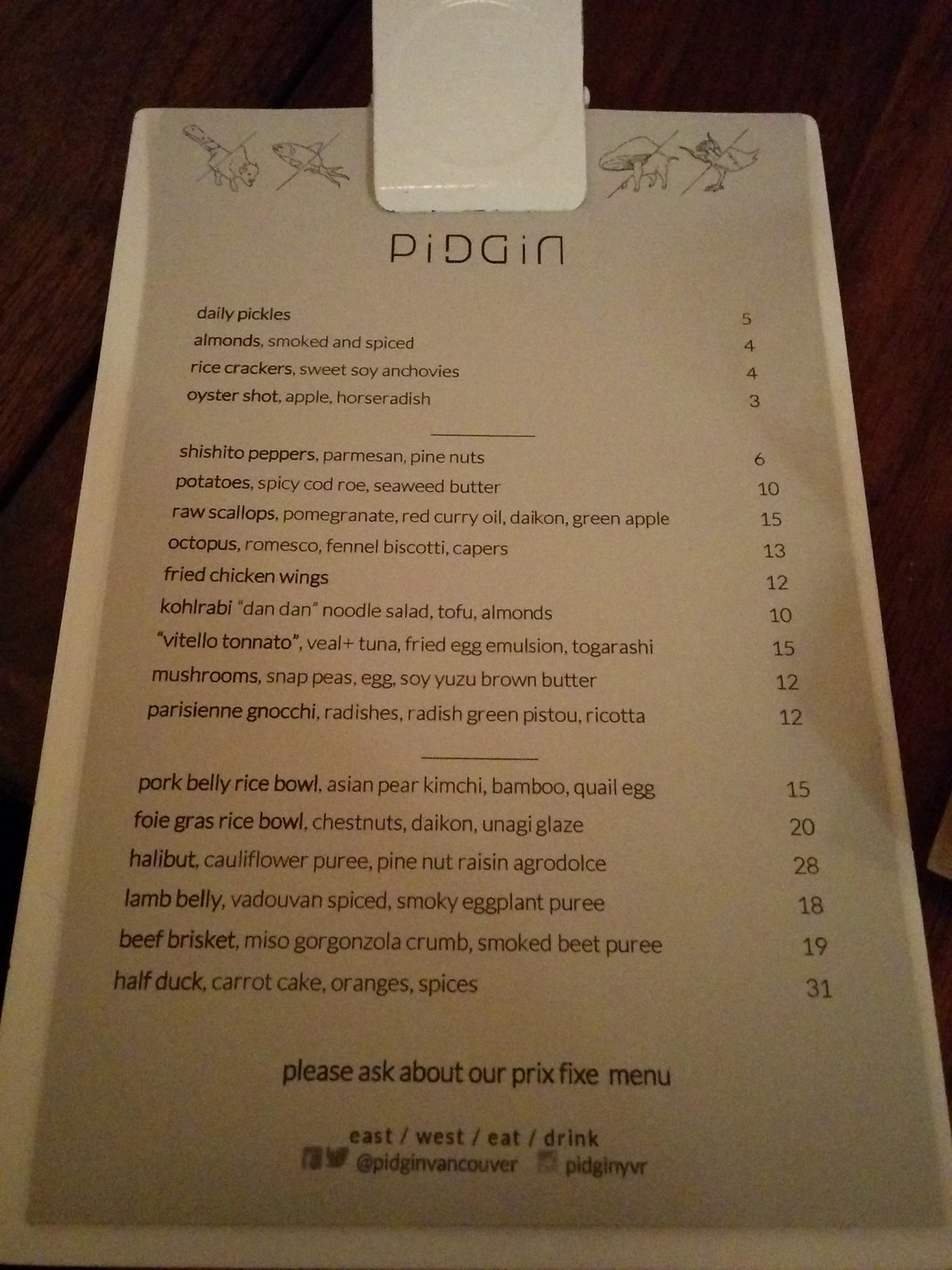Menu for Pidgin Restaurant (P-I-D-G-I-N)

- Daily Pickles: $5 
- Smoked and Spiced Almonds: $4 
- Rice Crackers with Sweet Soy and Anchovies: $4 
- Oyster Shot with Apple and Horseradish: $3 
- Shishito Peppers with Parmesan and Pine Nuts: $6 
- Potatoes with Spicy Cod Roe and Seaweed Butter: $10 
- Raw Scallops with Pomegranate, Red Curry Oil, Daikon, and Green Apple: $15 
- Octopus with Romesco, Fennel Biscotti, and Capers: $13 
- Fried Chicken Wings: $12 
- Kohlrabi Dan Dan Noodle Salad with Tofu and Almonds: $10 
- Vitello Tonnato (Veal and Tuna) with Fried Egg Emulsion and Togarashi: $15 
- Mushrooms with Snap Peas, Eggs, Soy, and Yuzu Brown Butter: $12 
- Parisian Gnocchi with Radishes, Radish Greens, Pistou, and Ricotta: $12 
- Pork Belly Rice Bowl with Asian Pear, Kimchi, Bamboo, and Quail Egg: $15 
- Foie Gras Rice Bowl with Chestnuts, Daikon, and Unagi Glaze: (Price not listed)
- Halibut with Cauliflower Puree, Pine Nut Raisin, and Agrodolce: $28 
- Lamb Belly with Vadouvan Spice, Smoky Eggplant Puree, Beef Brisket, Miso, Gorgonzola Crumb, Smoked Beef Puree, Half of a Duck: $31 
- Carrot Cake with Oranges and Spices: (Price not listed)

Please inquire about our prix fixe menu, East-West Eat and Drink.

Follow us on Instagram:
- Pidgin Vancouver
- PidginYVR